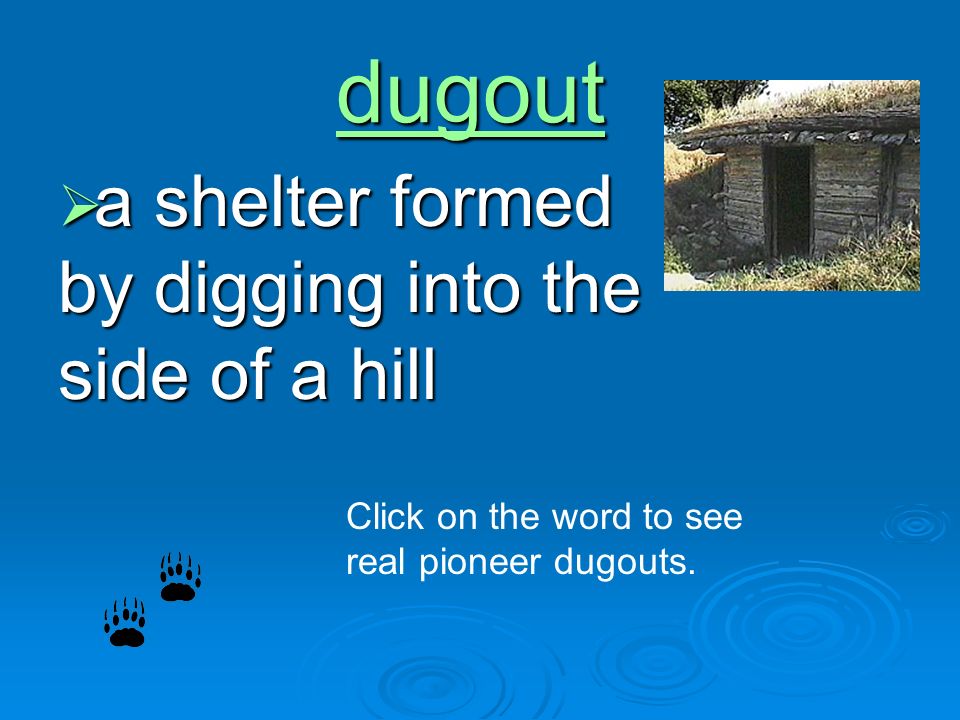The image appears to be a page from a textbook or online educational material about various forms of home architecture across different cultures and historical periods. The entire slide has a blue background that transitions from lighter blue at the bottom to a slightly darker blue at the top. In the lower right section, there are water ripple patterns, resembling the effect of a pebble being dropped into water, with at least four such patterns created by oval rings. Additionally, the bottom left corner contains two small, black bear paw prints.

At the top of the slide, in green, underlined, Comic Sans-like text, the title "dugout" is displayed. Beneath this title is a bullet point represented by a green and blue arrow pointing to the right. The accompanying text, in white and lowercase except for a capital "C" in "Click," reads: "a shelter formed by digging into the side of a hill." Further down, in smaller light blue text, it says: "click on the word to see real pioneer dugouts."

On the top right corner of the slide, there is a rectangular photograph approximately 3 cm tall by 7 cm wide, showcasing an example of a dugout shelter. This shelter appears to be a low log structure with an open, doorless entrance. The roof is covered in dry grass and dark wood, and there are trees with green foliage visible in the background, along with green grass in the foreground, denoting a natural setting.